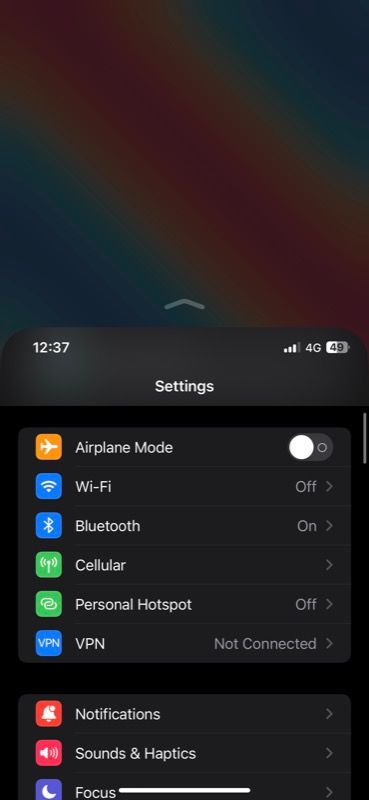The image displays a cell phone screen showing a variety of system status indicators and settings. The time on the phone is 12:37, and the device has 4G connectivity with three bars of signal strength. Airplane mode is enabled, as indicated by the switch being slid to the on position. Wi-Fi is turned off, while Bluetooth is active. The cellular data option has not been accessed, leaving it closed. The personal hotspot feature is disabled, and the VPN is not connected.

The background of the phone screen is predominantly black with a colorful, rainbow-like gradient running diagonally from the northwest to the southeast corner. Located beneath the primary settings (Airplane Mode, Wi-Fi, Bluetooth, Cellular, Personal Hotspot, VPN) is a blank bar, followed by a section labeled "Notifications," which is not expanded. Further options shown on the screen include "Sounds & Haptics" and "Focus," each represented by icons - with "Focus" illustrated by a crescent moon. Neither of these sections is opened. The overall interface suggests this is the settings menu of the phone.